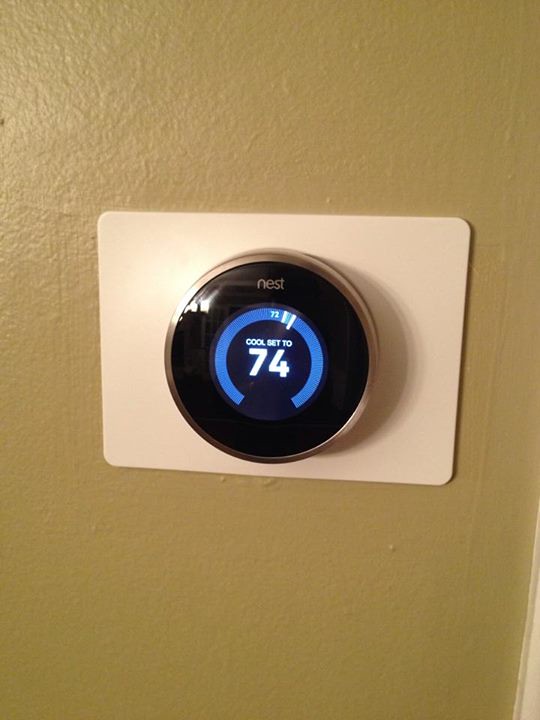In this photograph, a Nest smart thermostat is mounted on a mustard yellow wall. The thermostat sits on a white plastic backing that is rectangular and slightly larger than the device itself, providing a subtle contrast between the sleek circular gadget and the vivid wall color. The digital display on the Nest thermostat is lit, indicating that it is currently set to cool the room to 74 degrees Fahrenheit. A semi-circle light blue bar surrounds the "cool set to 74" text, visually signifying the cooling mode. Soft light from an external source illuminates the scene from the left, adding a gentle glow to the overall composition.